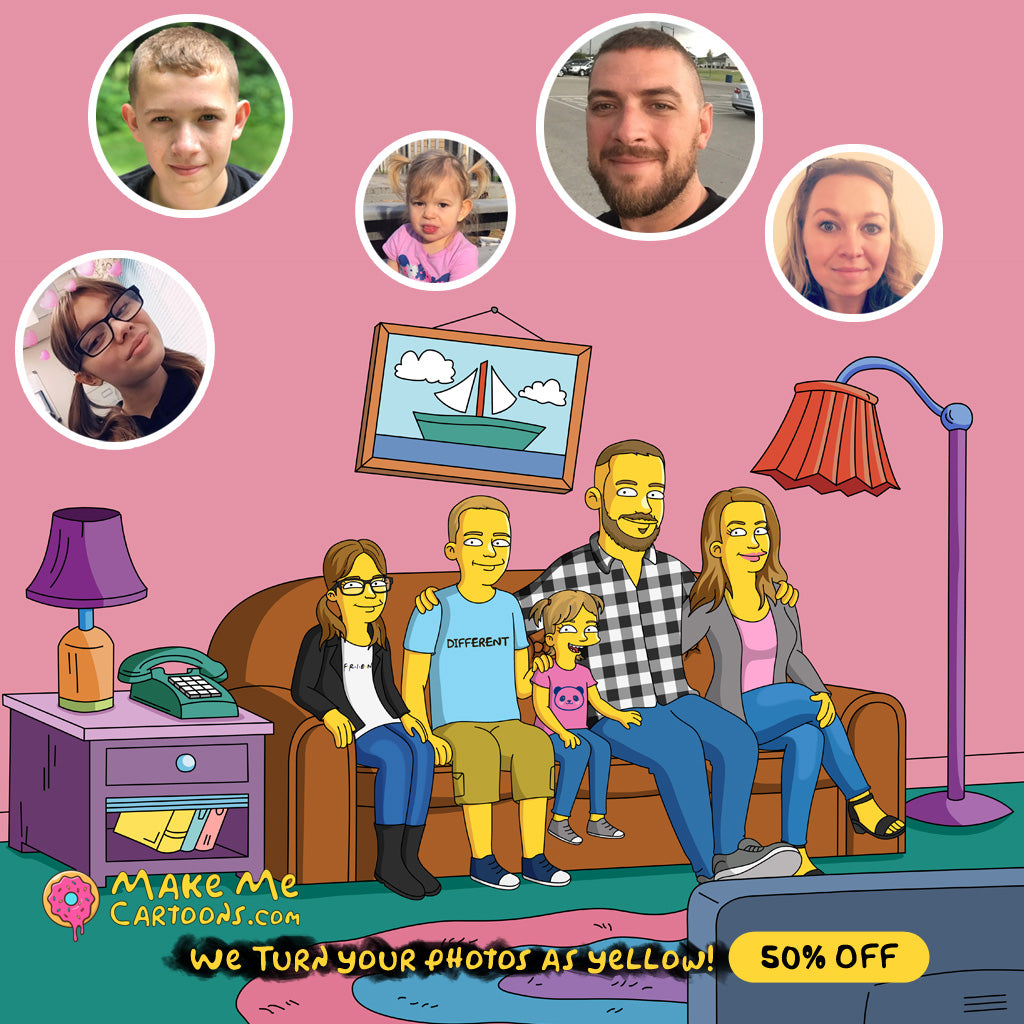An advertisement from MakeMeCartoons.com features a whimsical image where a family of five is transformed into yellow-skinned cartoon characters reminiscent of "The Simpsons." The company's logo, a pink frosted donut, sits prominently at the top against a soft pink background. The advertisement shows individual photographs of the family members—a father, mother, teenage girl, younger boy, and a baby—each encased in a white circular frame above the cartoonized versions. In the illustration, the family is seated on a couch, with the father's beard, the girl's glasses, and their clothing accurately mirrored from the real photos. Surrounding the cartoon family are various household elements: a purple end table adorned with a purple lampshade lamp and a green push-button telephone, as well as a crooked picture of a sailboat above the couch. Beneath this playful family portrait, text reads "MakeMeCartoons.com" followed by "We turn your photos as yellow!" in bright yellow lettering against a black backdrop, highlighting a tempting "50% off" offer.